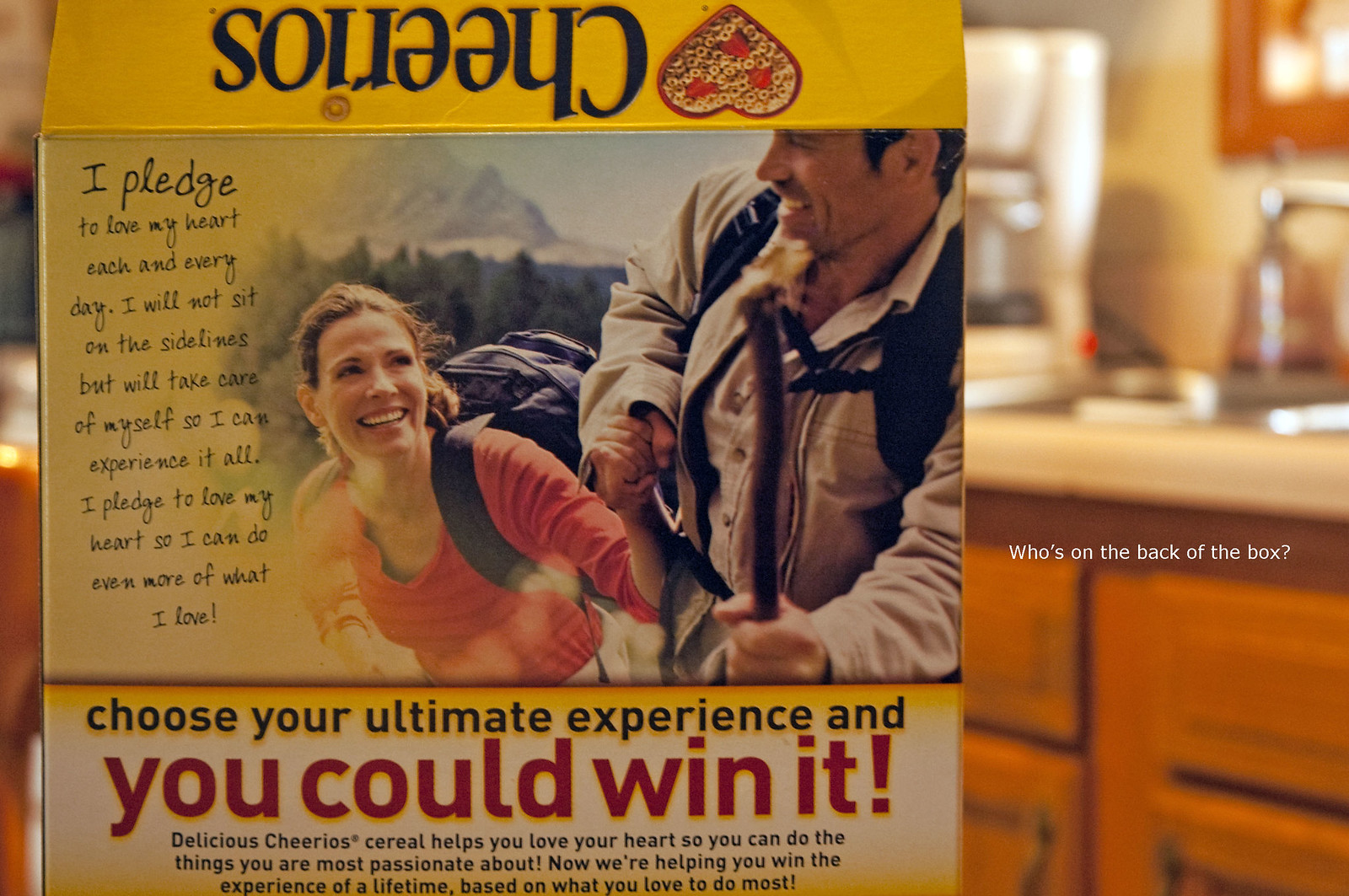This image displays the back of a yellow Cheerios cereal box, set against a blurred kitchen background featuring cabinets, a countertop, a coffee maker, and a sink. Prominently featured at the top of the box is the upside-down Cheerios logo, accompanied by a heart-shaped red bowl filled with cereal and strawberries. Below this, a clear image showcases a smiling man and woman, both wearing backpacks and appearing to be hiking in a mountainous area. 

Central to the box is bold text encouraging engagement: "Choose your ultimate experience and you could win it," with "you could win it" highlighted in red. Additional supportive text in black beneath emphasizes the nutritional benefit: "Delicious Cheerios cereal helps you love your heart so you can do the things you're most passionate about. Now we're helping you win the experience of a lifetime based on what you love to do most."

Another notable section features a personal pledge in smaller black text: "I pledge to love my heart each and every day. I will not sit on the sidelines but will take care of myself so I can experience it all. I pledge to love my heart so I can do even more of what I want." Overlaying the kitchen cabinets in white text, it reads: "Who's on the back of the box?"

Overall, the detailed depiction on the Cheerios box combines both visual and textual elements focusing on heart health, outdoor adventures, and the potential to win an experience based on personal passion.